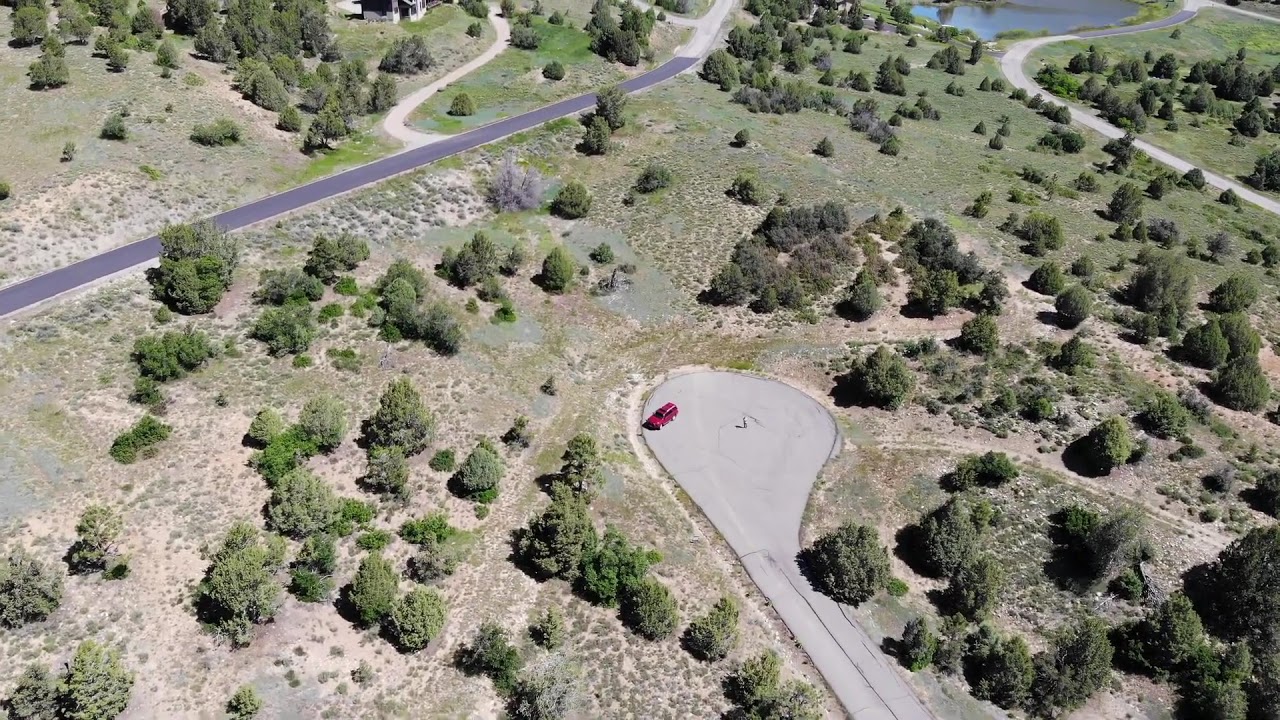The aerial image depicts a piece of land scattered with green trees and dry grass. Near the top left corner, a narrow grey road extends diagonally, branching into lighter-colored paths that penetrate deeper into the green landscape. The top right corner features another narrow road winding around a small body of water. Dominating the center, a circular cul-de-sac connects to a straight road that leads downwards to the bottom of the image. Parked in the center of this roundabout is a lone red minivan or SUV. Surrounding the cul-de-sac is dense brush and trees, with the overall terrain appearing dry and sparsely vegetated.